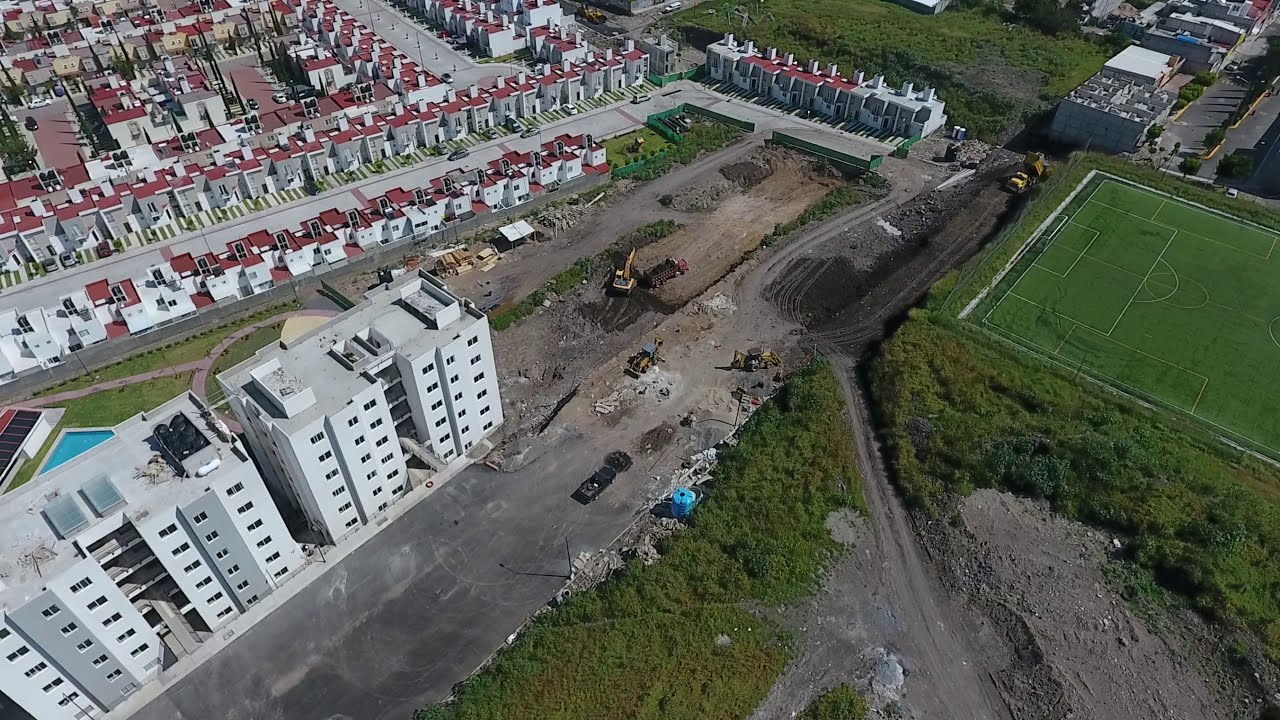The image reveals a top-down aerial photograph of a sprawling suburban area interspersed with construction and recreational zones. In the foreground, there's a large multi-story white building, seemingly under construction, evidenced by heavy machinery and dirt lanes surrounding a partially developed parking lot. Behind this structure, a chain of identical white homes with reddish roofs stretches out, forming neat subdivisions, intersected by gray concrete roads. Further in the background, a substantial blue triangle hints at the edge of a large swimming pool. Off to the side, the photograph captures a vast green soccer field, marked vividly with white lines. The right edge of the image shows grassy areas, contrasting with the uniformity of the residential sections, concluding with additional buildings in the top right corner. The entire scene conveys a blend of developed residential areas and active construction zones, suggesting ongoing expansion.